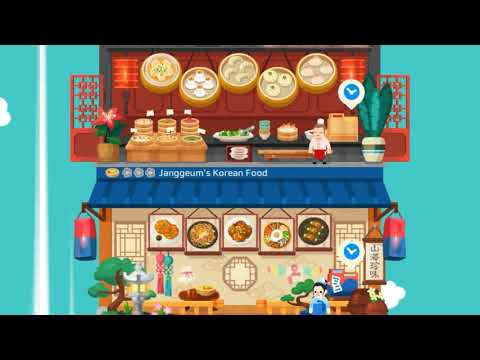The image is a vibrant scene from a video game, showcasing a bustling, multi-tiered marketplace inspired by Japanese and Korean cultures. The upper section of the scene resembles a Japanese restaurant adorned with deep reddish walls. Circular bowls filled with various dishes are arrayed on tables, alongside decorative plants and flowers, all set against a teal blue background with fluffy clouds. Screens flank the tables, providing a traditional ambiance.

The middle section features a prominent roof structure inscribed with the name "Janggyum's Korean Food" in blue and white writing. Below this sign, a Korean restaurant with a blue-roofed stall displays several tantalizing food pictures. A sign in Korean is visible on the right side, next to a red and blue cash register. To the left, a person stands amid the decor, which includes bonsai trees and traditional screen dividers, and two hanging lanterns.

Every detail, from the lush plants to the meticulous arrangement of food items and cultural decor, creates an immersive and lively atmosphere, drawing players into this culinary-themed virtual world.